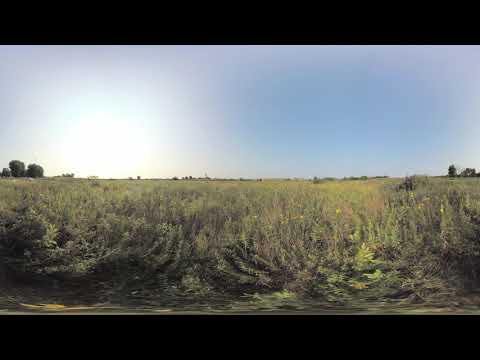This image captures a vast, flat, overgrown grassy field that resembles a prairie or a meadow. The field stretches out with various shades of green from the underbrush, tall grasses, and sparse shrubs. In the distance, along the horizon, faint and far-off trees can be seen dotting the landscape. The sky above is a clear, bright blue with no clouds, and it's dominated on the left side by a large, glowing orb of the sun, casting hues of yellow, white, and orange light across the scene, indicating the time is around afternoon. The top and bottom parts of the image are bordered in solid black. The image's panoramic nature slightly distorts and curves the bottom, enhancing the expansive feel of this serene, sunlit outdoor setting.